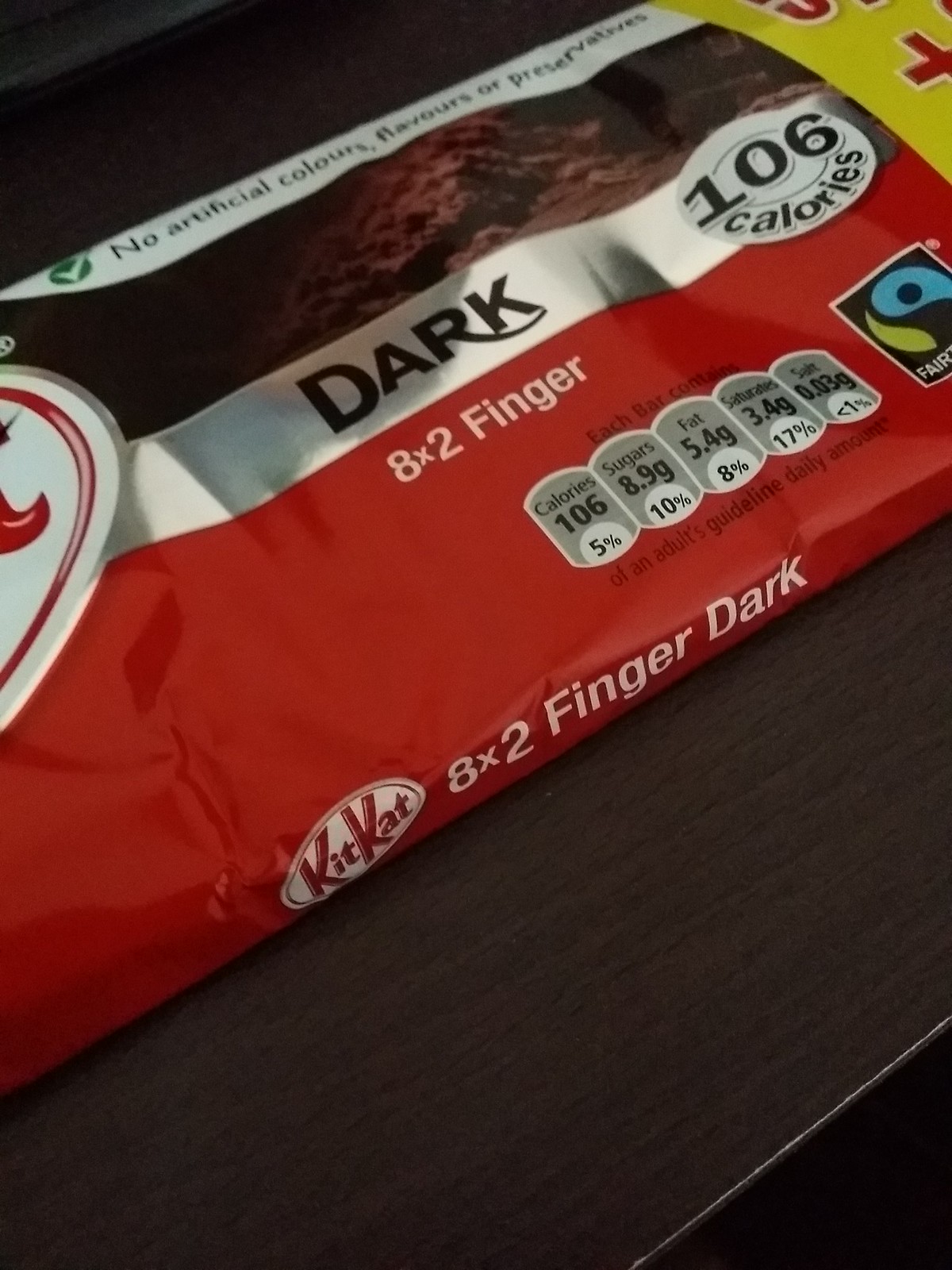The image features a partially visible bag of KitKat Dark Chocolate candy bars. The central section of the package prominently displays the text "Dark" and "106 Calories" in black ink on a white background. Below this, it reads "8x2 Finger." On the side, the iconic KitKat logo is shown in red letters with a white oval background, alongside the notation "8x2 Finger Dark" in white letters. The top of the package contains a statement in favor of natural ingredients, reading "No Artificial Colours, Flavours, or Preservatives," with British English spellings indicating it might be a European product. The bottom right corner features a green and blue logo on a black background, signifying Fairtrade certification. Nutritional information is also provided: each bar contains 106 calories, 8.9 grams of sugar, 5.4 grams of fat, 3.4 grams of saturated fat, and 0.03 grams of salt.